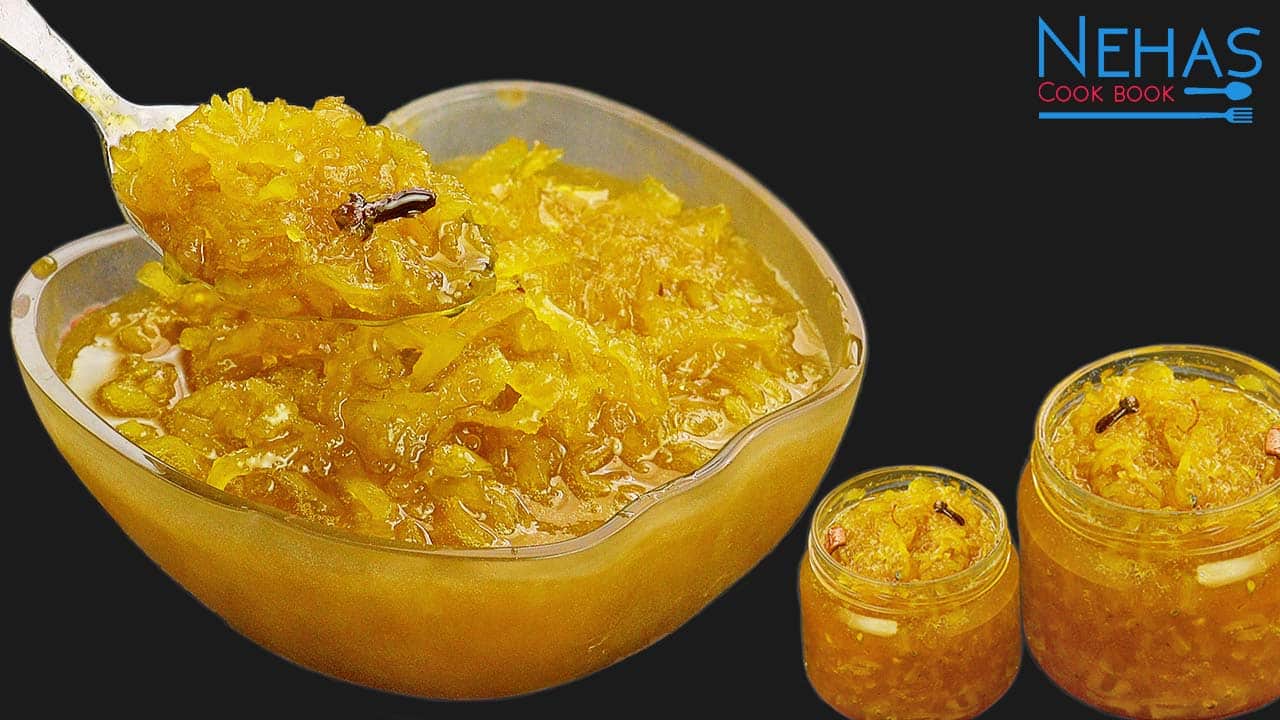In this striking black-background photograph from "Neha's Cookbook," a crystalline, apple-shaped glass bowl glistens, filled with a vibrant, yellow, juicy concoction that exudes a slightly slimy texture. This preserved food, possibly containing cloves or shredded yellow vegetables, is being lifted by a spoon, which shows remnants of the food and juice, hinting at its luscious consistency. Beside the main dish, two smaller glass containers, one larger than the other, are also packed with the same yellow mixture, their transparent walls revealing the food inside. Above, the elegant "Neha's Cookbook" logo is displayed in the upper right corner, featuring a drawn spoon and a long fork, which elegantly underline the text. The meticulous presentation emphasizes the contrast between the bright yellow food and the dark backdrop, making the dish visually pop.